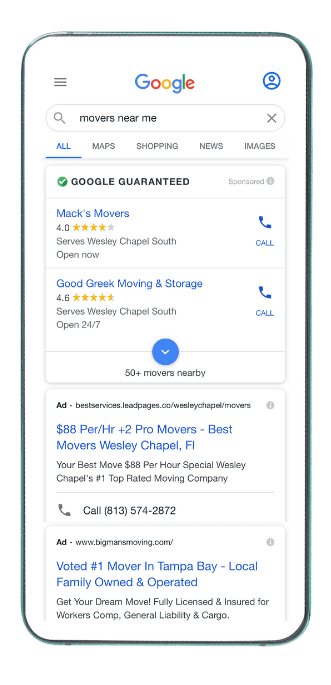The image displays an iPhone screen with a distinctive greenish and purplish outline. The screen background is white, and at the top left corner, there are three black horizontal lines. In the center, the Google logo is prominently featured, flanked by a blue circle containing additional blue circles within it. Below this, a white oval contains a gray magnifying glass icon followed by a text entry field, currently populated with the phrase "movers near me."

Just below this search bar, a series of tabs are visible: the "All" tab, highlighted in blue and underlined, the "Maps," "Shopping," "News," and "Images" tabs appear in black text. Directly beneath these tabs, a white box with a green circle beside it states "Google Guaranteed."

The search results display the following:

1. **Max Movers**:
   - Rating: 4.0 (displayed with four stars out of five)
   - Service area: Wesley Chapel South
   - Status: Open now
   - A blue "Call" link with a phone icon and the word "Google" above it

2. **Good Greek Moving & Storage**:
   - Rating: 4.6 (displayed with four and a half stars out of five)
   - Service area: Wesley Chapel South
   - Status: Open 24/7
   - A blue "Call" link with a phone icon

An additional note indicates more options with "50+ movers nearby" in black text accompanied by a downward-pointing blue arrow.

A highlighted advertisement at the bottom features the following details:
- Price: $88 per hour
- Service: Two professional movers included
- Claim: "Best movers in Wesley Chapel Hill"
- Slogan: "Your best move"
- Contact: $88 per hour special, Wesley Chapel's number one top-rated moving company
- Phone number: 813-574-2872